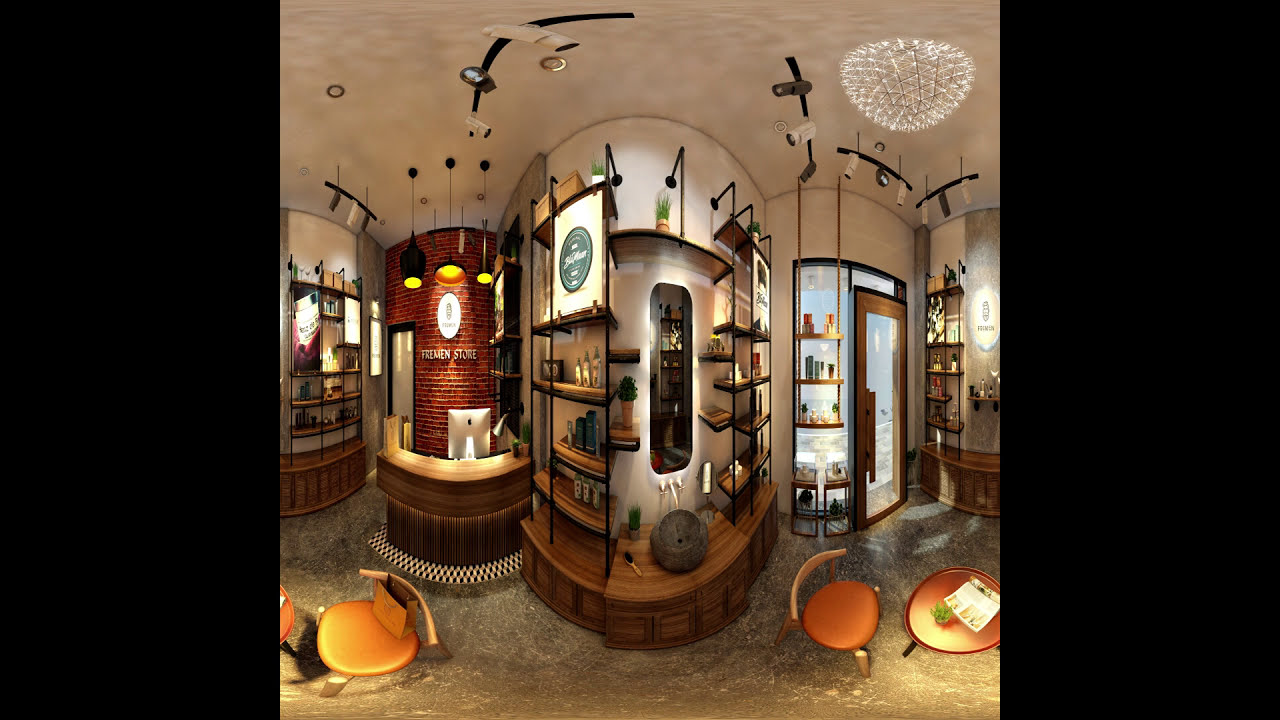This panoramic image showcases the interior of a high-end boutique, likely specializing in beauty or haircare products. Dominating the background is an exposed red brick wall featuring the store's logo "Freeman's Store" in gray letters. The store has a chic, sophisticated ambiance, characterized by a combination of both modern and rustic elements. 

On the brick wall, wooden shelves with a sturdy wooden base neatly display an assortment of bottles, likely premium haircare or beauty products, reinforcing the boutique's upscale nature. A little desk with a contemporary computer setup indicates the checkout or customer service area, next to which lies a brown wood countertop with a light brown top. The floor beneath features a striking black-and-white checkered pattern, transitioning into an overall gray tone.

Further inside, the boutique reveals more intricate details: crystal chandelier balls hanging from a pristine white ceiling cast a warm, yellow glow over the scene. The furnishing includes uniquely designed brown chairs with white-brown backs, and cherry wood tables. One table prominently displays a green plant and an open magazine or paper. 

On the left side of the image, another glass display case with shelves holding various bottles is seen, possibly lotions. Near this, peculiar, contoured chairs are angled oddly due to the panoramic distortion but add to the boutique's bespoke décor. All these details contribute to an impression of luxury, making it evident that the boutique is potentially part of an upscale salon offering exclusive haircare products.